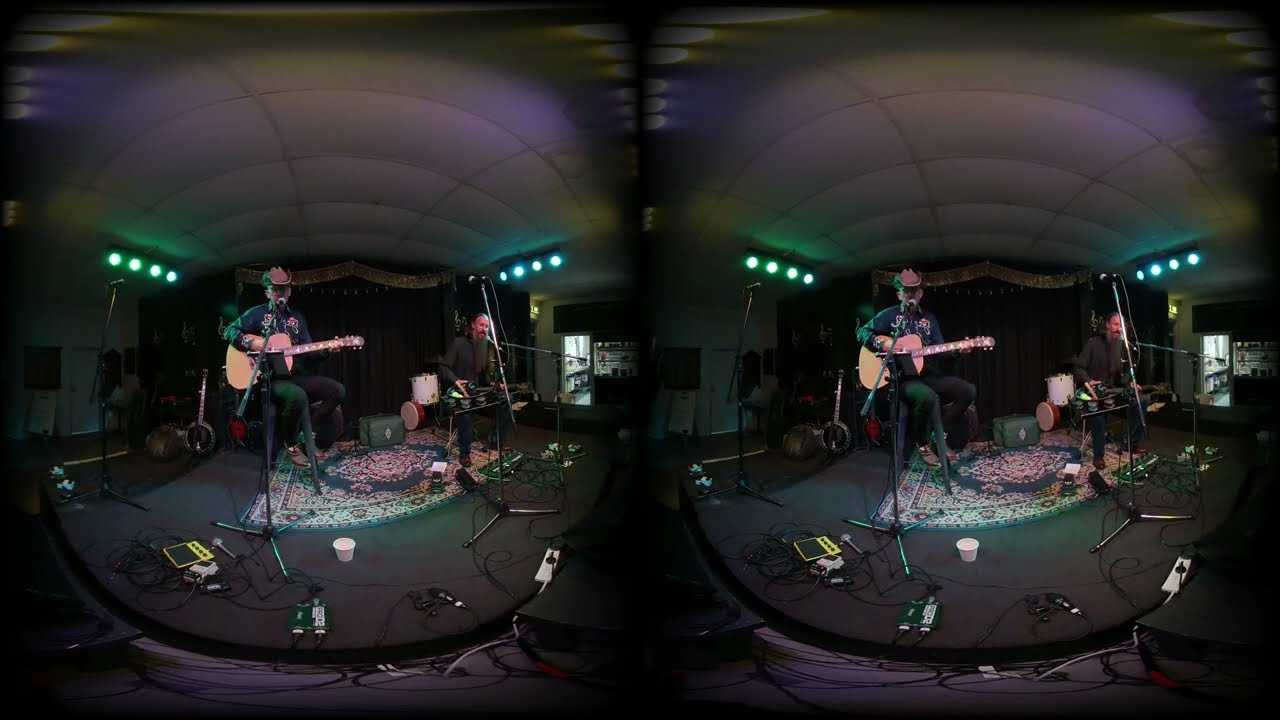The image features a horizontally split, rectangular photo showing two slightly warped, fish-eye views of the same scene, creating a panoramic effect. The main subject is a man standing at a microphone, holding a brown guitar and singing, dressed in a black long-sleeve shirt, blue jeans, and a cowboy hat. He stands on an ornate blue and red rug, with a thin, dark blue-gray carpet beneath it. In the background to the right, another man is visible, possibly seated or standing at a keyboard, also equipped with a microphone. The scene appears to be set in a recording studio or staged area, with additional musical equipment visible, including speakers, other microphones, a banjo, and what might be some drums, although there's no drummer present. The backdrop includes curtains, likely covering a stage, with white ceilings and lights on either side. The entire scene is rich in detail, capturing the essence of a live musical setup.